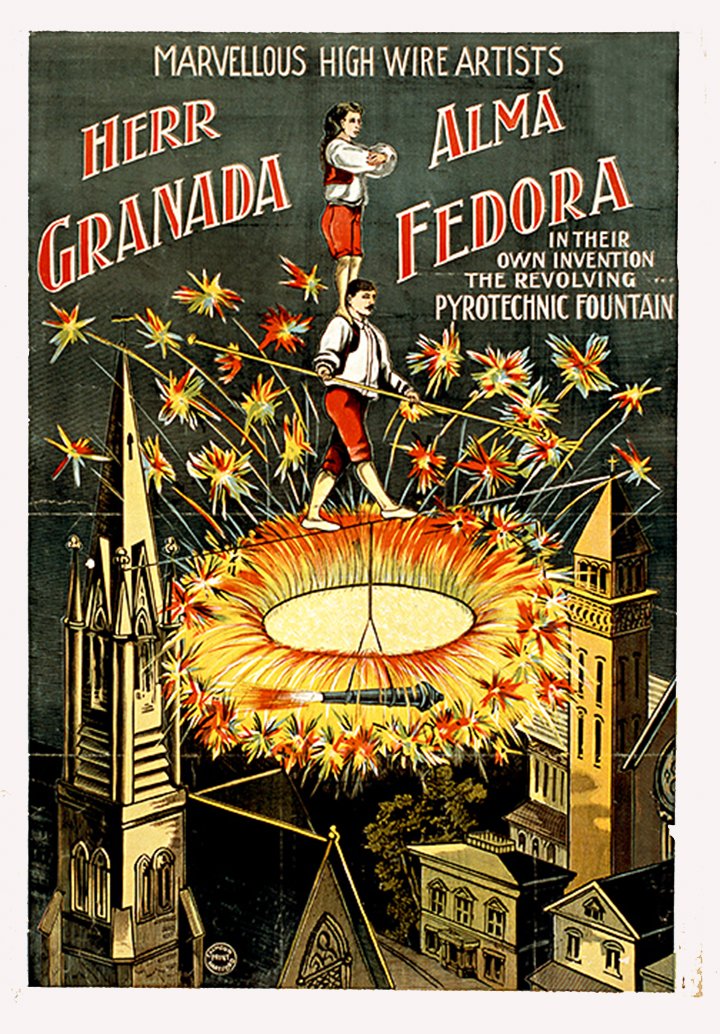The image is a vintage poster advertising a high wire act featuring Marvelous High Wire Artists, Her Granada and Alma Fedora. The centerpiece of the illustration depicts a daring scene where a man in red pants and a white shirt is walking a tightrope stretched between a cathedral and another tall clock tower. Balancing on his shoulders is a woman dressed in red shorts and a white shirt, gripping his shoulders for stability. The man steadies himself with a long brass rod. Surrounding them is a spectacular pyrotechnic display—fireworks bursting in all directions from a revolving ring below them, termed their own invention: the "Revolving Pyrotechnic Fountain." The background showcases the roofs and facades of the two tall buildings, adding to the dramatic height and risk of the act. The top of the poster reads in bold, white letters, "Marvelous High Wire Artists," while below, red lettering on a white board announces "Her Granada and Alma Fedora," emphasizing the grandeur and innovation of their performance.